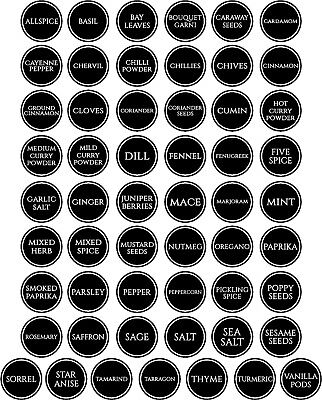This is a detailed black-and-white image featuring a grid of 55 circular spice stickers, designed in alphabetical order. Each sticker represents a spice name, with a black background, a thin white circular outline, and prominently displayed white block lettering in the center. The grid is composed of 8 rows of 6 stickers each and a final row containing 7 stickers. The background is entirely white, emphasizing the contrast with the black stickers. The spice names vary, including allspice, basil, bay leaves, caraway seeds, chili powder, cinnamon, cloves, cumin, dill, fennel, ginger, juniper berries, mace, mustard seeds, nutmeg, pepper, poppy seeds, sage, sea salt, sesame seeds, smoked paprika, star anise, tarragon, thyme, vanilla pods, and many others. The text size on each sticker adjusts according to the length of the spice name, ensuring all names fit neatly within the circular space. This meticulously arranged design likely represents spice jar lids or labels.